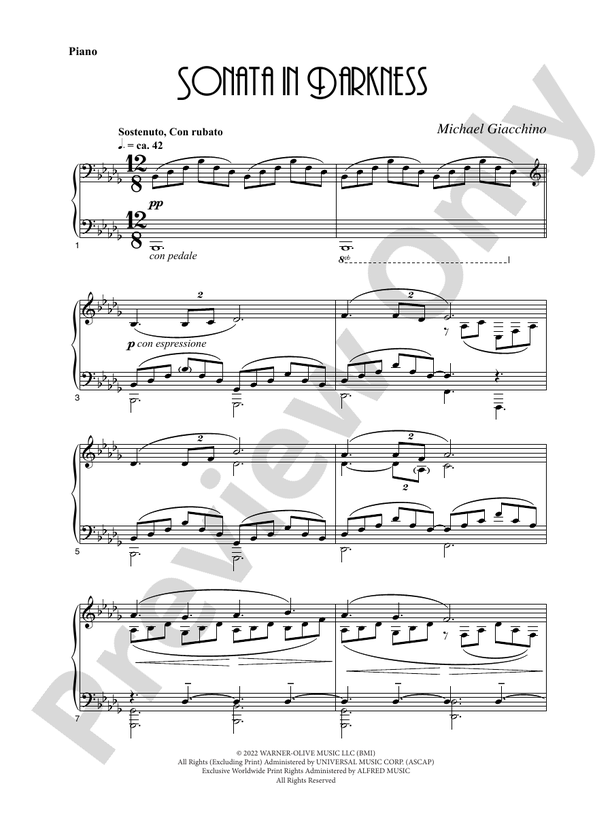This detailed image features a sheet of piano music for "Sonata in Darkness" by Michael Giacchino. The sheet is watermarked with "preview only," indicating it's a preliminary version. Published in 2022 by Warner Olive Music LLC (BMI), with all rights excluding print administered by Universal Music Corp (ASCAP) and exclusive worldwide print rights managed by Alfred Music, all rights are reserved. The sheet displays the musical notation and terms essential for performing the piece, including key signatures and time signatures like 12/8.